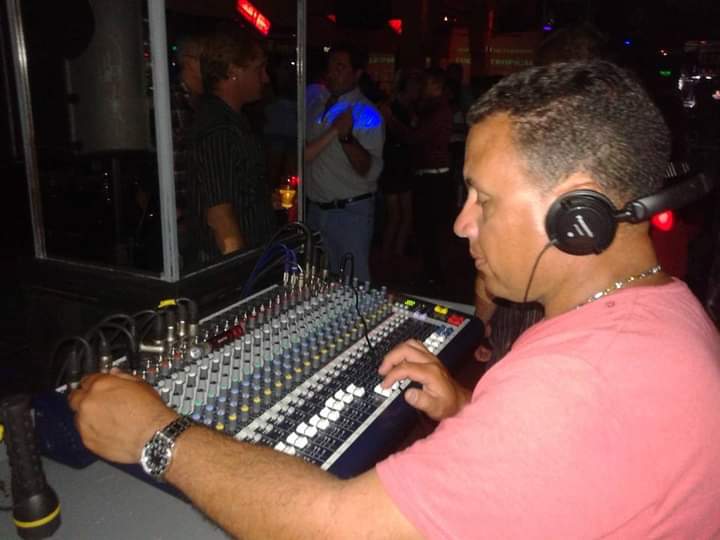The photograph captures a DJ, likely of Hispanic descent, in the midst of his performance at a club or bar. The DJ is shown in a side profile, looking to the left, with his eyes closed or partly open, immersed in his task. He sports a salmon-colored, short-sleeved shirt, black headphones over his short dark brown hair, a silver wristwatch on his left wrist, and a silver necklace around his neck. The DJ is seated in front of a complex control panel filled with numerous buttons, knobs, and wires. His left hand is adjusting a setting while his right finger is pushing a button. A black flashlight is positioned on the left-hand side of the panel. The background is dimly lit with dark colors punctuated by vibrant blue and red lights from the ceiling. Several people are faintly visible, including a man with blonde hair and a green and silver striped shirt standing closest to the DJ. There's a mirrored pole and what seems to be a bar area with people milling around and chatting, adding to the lively atmosphere of the scene. The overall palette includes shades of brown, black, tan, white, pink, yellow, blue, and red, reflecting the dynamic and colorful environment.